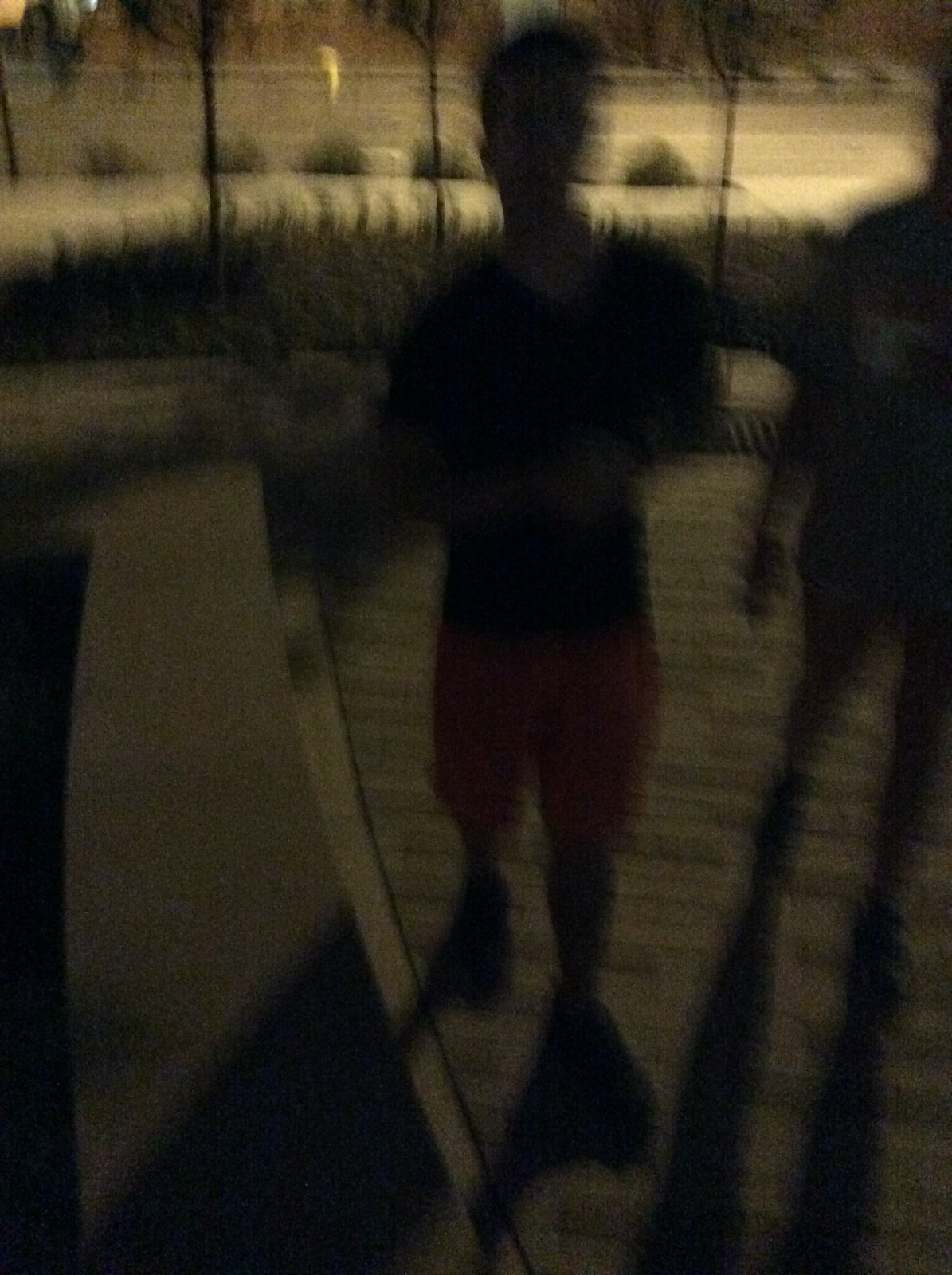In this blurry outdoor image, two individuals are depicted. The first person, who is fully visible, appears to be male and is dressed in pink or red shorts with a black shirt, and might be wearing a watch on his wrist. The second person is partially visible, with just one arm and two legs showing, also dressed in shorts. To the left of them stands a bench. Behind the pair lies a parking lot, accompanied by some bushes and trees. They are walking along a brick walkway.